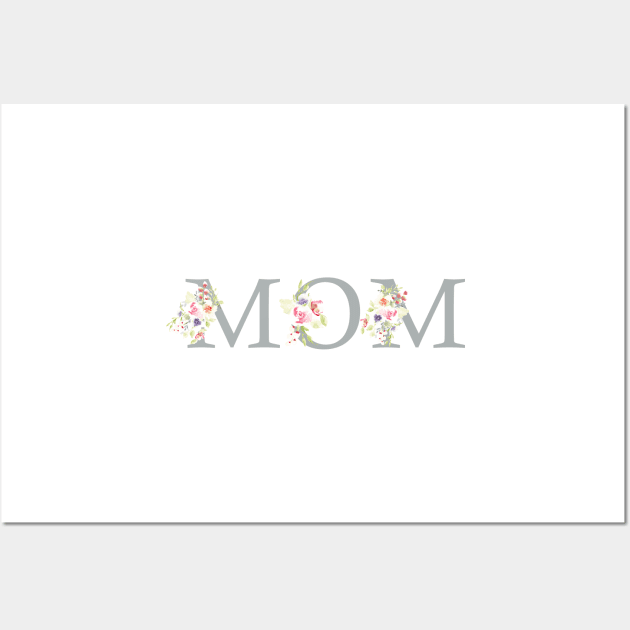This image depicts a minimalist digital illustration with a light gray background. At its center is a white rectangle, subtly shadowed on the bottom and right sides to create a slight three-dimensional effect. Dominating the center of this rectangle is the word “MOM,” written in large, medium-gray serif font. Each letter features a decorative flourish on its left side, where clusters of flowers appear to merge into the letters, suggesting a disintegration into blossoms. These clusters, likely resembling watercolor roses in varying shades of red, pink, and purple, are interspersed with delicate light green and yellow leaves, and accented with small red dots. The floral designs, each slightly distinct, present an elegant touch that complements the serif text, filling the left upper and diagonal lines of both "M"s, and the left side of the "O". The refined and flat design, indicative of digital artwork, is set against a plain white background enclosed by a thin, light gray outline, adding to the image's clean and sophisticated look.